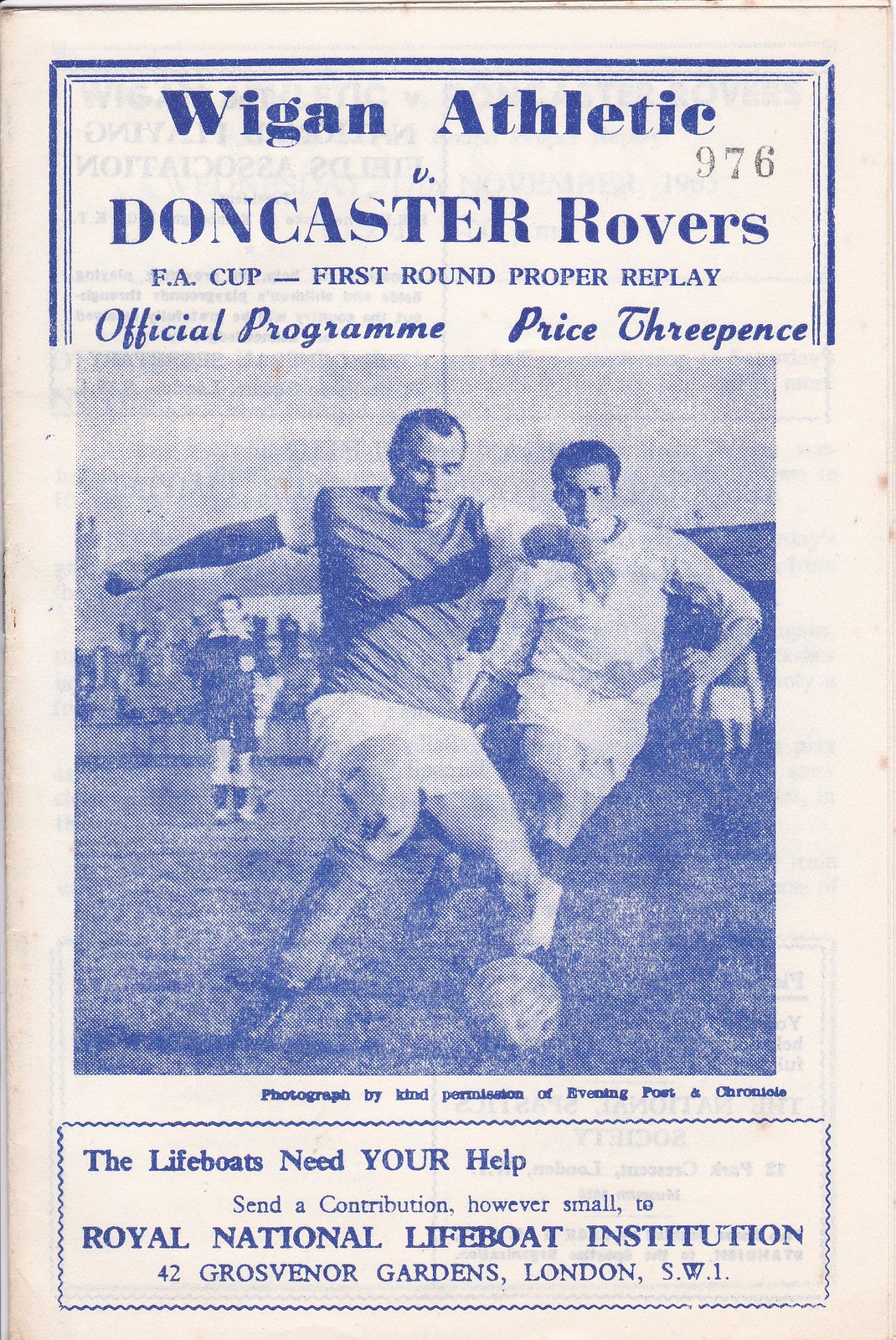The image showcases an aged pamphlet, likely a page from a soccer program or brochure, predominantly featuring a blue theme. At the top, within a small blue-bordered box, it reads "Wigan Athletic" in bold, followed by "versus Doncaster Rovers" and the number "976" to the right. This is described as the "FA Cup first round proper replay." Below, the text "Official Program" and "Price 3 Pence" are written in cursive. Dominating the center is a black-and-white photograph of soccer players; in the foreground, a player in a lighter uniform (likely white) is about to kick the ball with his left foot, arms spread out for balance. Another player in a darker shirt with white shorts is seen running toward the ball. Additional players can be glimpsed in the background. Below the photograph, it notes that the image is published "by kind permission of the Evening Post and Chronicle." At the bottom, the pamphlet appeals to readers with, "The Lifeboats need your help. Send a contribution, however small, to Royal National Lifeboat Institution, 42 Grosvenor Gardens, London SW1."